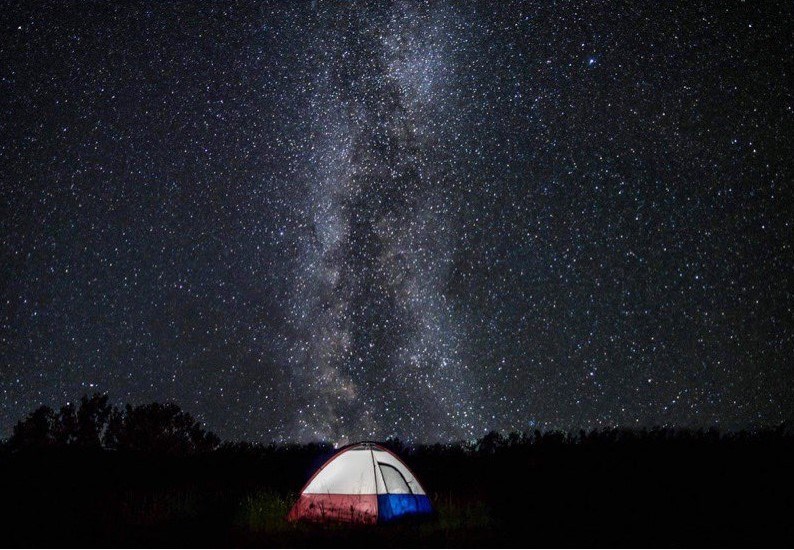The image captures a vibrant camping scene in the dead of night, showcasing a lit-up tent. The tent is predominantly white on top with a red section on the bottom and side, and a blue section on the right where the entrance is, which is outlined in black. The tent is surrounded by an almost impenetrable darkness, obscuring the ground and creating silhouettes of trees that nearly match the tent's height, particularly on the left where some trees rise significantly higher. Moving right, the trees slope evenly higher than the tent. A striking night sky dominates above, filled with countless white, blue, and yellow stars. Notably, two bright white streaks stretched vertically through the center of the sky hint at a nebula, making it appear as though the tent glows almost as brightly as the stars themselves.